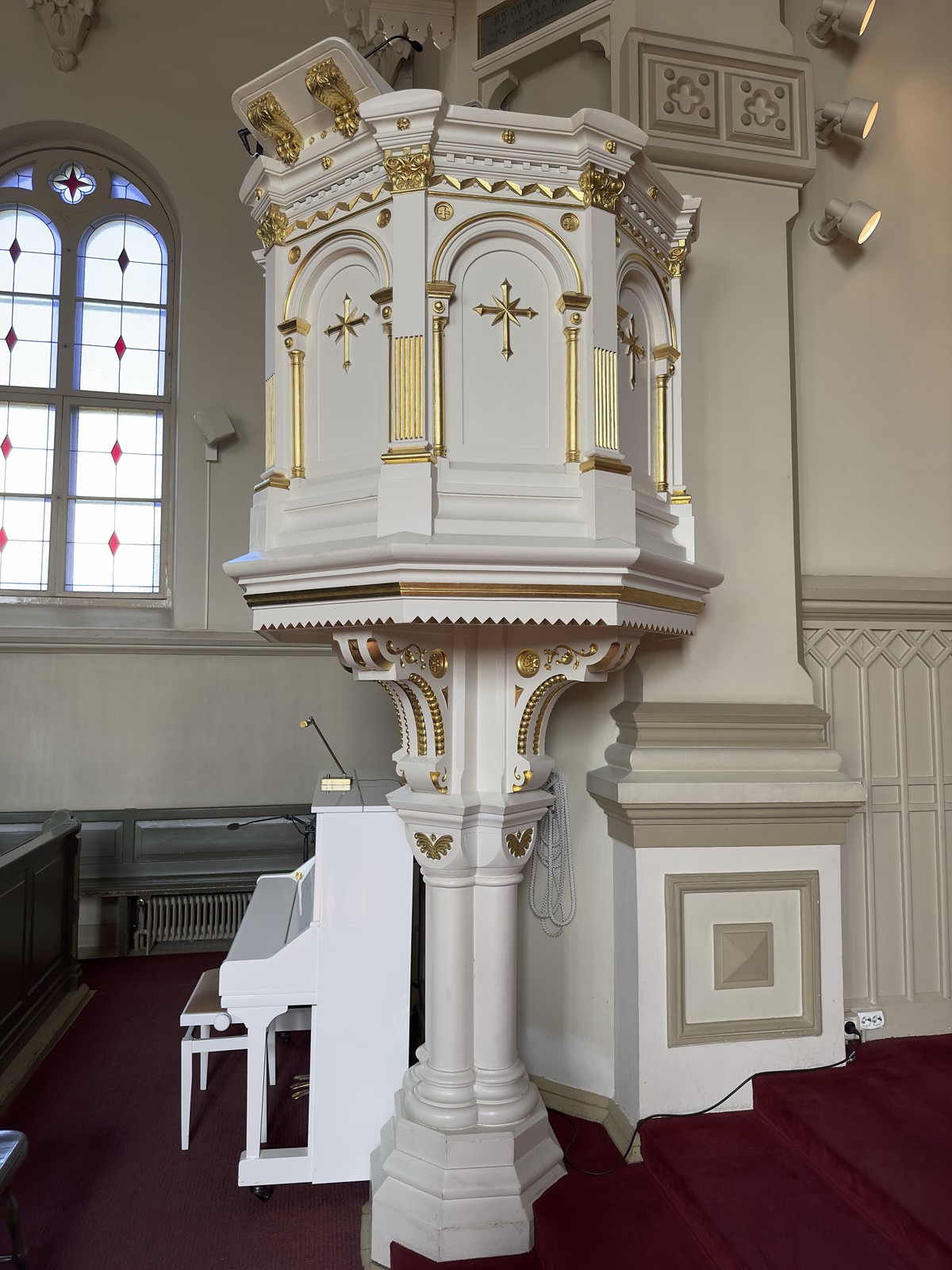The photograph captures the interior of an ornate, historic church. The composition highlights the church's elegant details. The walls are predominantly white, adorned with intricate gray moldings and decorative designs. A notable feature is the arched stained-glass window in the upper left corner, simple in design with white and red diamonds, adding a serene touch to the setting.

In the bottom left, the front of a brown wooden pew is visible, hinting at the traditional seating arrangement. Adjacent to the pew is an all-white piano, centrally positioned, lending a sense of purity and sophistication to the space. Dominating the scene is an elaborate, white carved pulpit or podium adorned with golden crosses and ornate decorations. This structure, open at the top, suggests a place where sermons or speeches would be delivered, despite the lack of visible steps leading up to it.

The floor is primarily covered with brown flooring, except for a section of rich red carpet on the lower right corner, leading up a set of low stairs lined in the same red carpet. This adds a touch of warmth and color contrast to the otherwise white-dominated interior. The overall atmosphere exudes a blend of reverence and grandeur, characteristic of a historic place of worship.